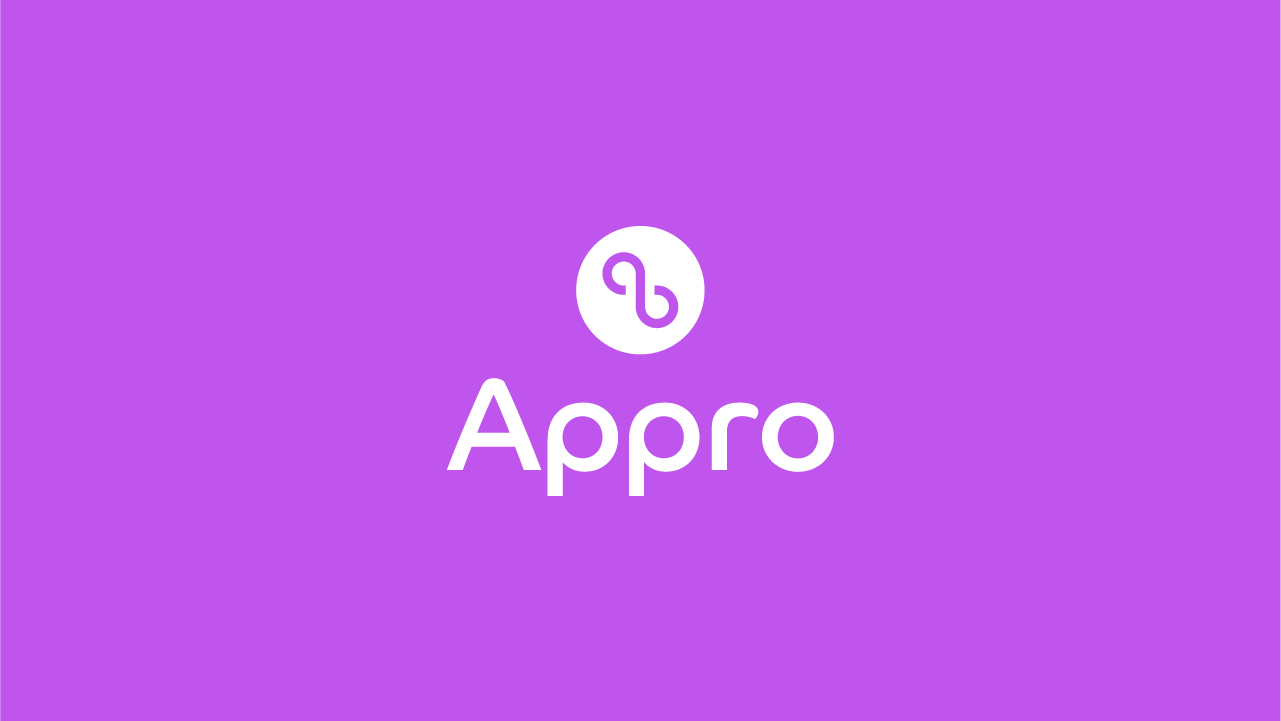The image features a horizontally oriented rectangle with a vibrant lavender background, leaning more towards a purplish-pink hue. Dominating the center of the image is the white text "APPRO," written in all capitals. Above the text is a distinctive white circular logo containing a broken, diagonally oriented infinity symbol. The simplicity of the design, highlighted by its two-color palette of purple and white, makes the details stand out against the bright background. The overall composition suggests it could be a logo page for a website or software application.